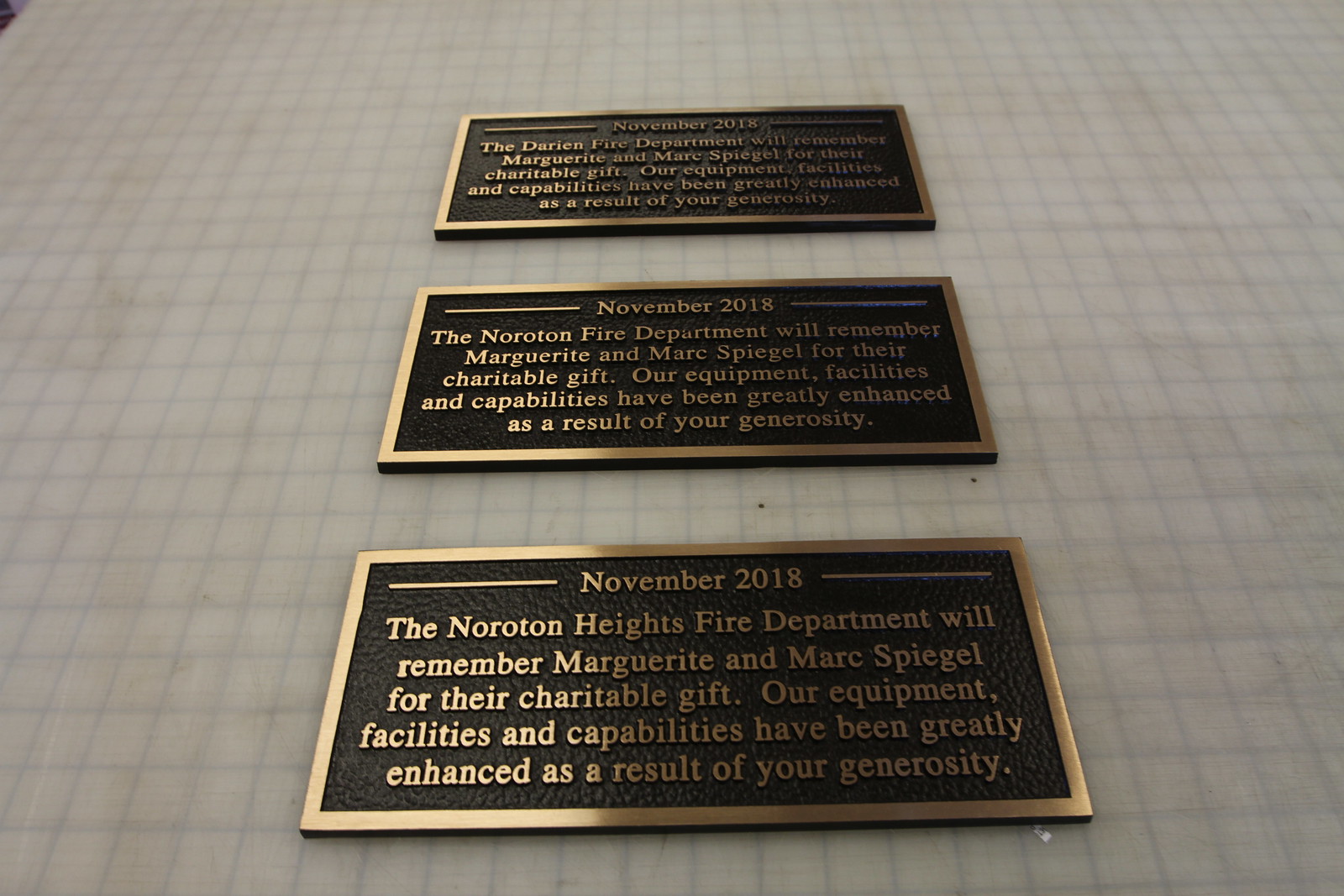In this indoor color photograph, we are presented with a white wall that has three brass plaques arranged vertically and equally spaced, set against a faint gray grid background that resembles graph paper. The brass plaques, each with polished rims and matte black backgrounds, feature identical text. They read: "November 2018. The Noroton Heights Fire Department will remember Marguerite and Mark Spiegel for their charitable gift. Our equipment, facilities, and capabilities have been greatly enhanced as a result of your generosity." The plaques are cast in bronze with raised lettering and a narrow border. The photograph is taken at a slight angle, making the plaque closest to the viewer appear larger. The right side of the plaques is partially shadowed, while the left side is more clearly illuminated, enhancing their legibility.